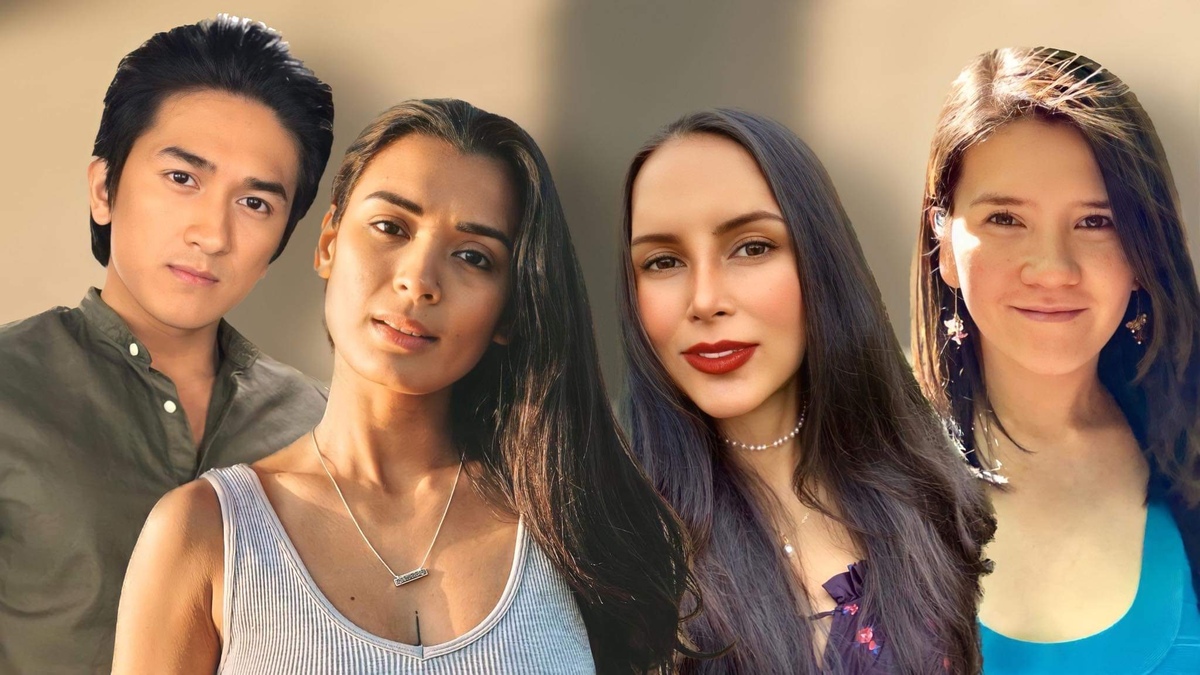In this detailed studio-captured image, four individuals stand in focus against a blurred background, likely as a cast for a show or movie. On the far left is an Asian man in his late 20s to early 30s with short, slicked-back jet black hair and dark eyebrows. He is wearing a greenish-gray button-up shirt with two buttons unbuttoned at the collar. Next to him is a Latina woman with olive skin, long dark brown hair, and dark brown eyebrows. She displays a slightly worried expression and is adorned with a silver necklace, wearing a ribbed white tank top. To her right stands another Latina woman with long, dark brown hair and lighter brown eyebrows, wearing bright red lipstick. She is slightly smiling, donning a small pearl necklace and a purple frilly t-shirt with pink flowers. On the far right is another Latina woman, also around 20 to 30 years old. She has lighter brown hair with very light eyebrows, minimal makeup, dangling earrings, and is wearing a blue shirt with a subtle, closed-mouth smile. The setup of the image, with its focus on the subjects and a blurry background, suggests a professional context, possibly highlighting themes of diversity and inclusion.